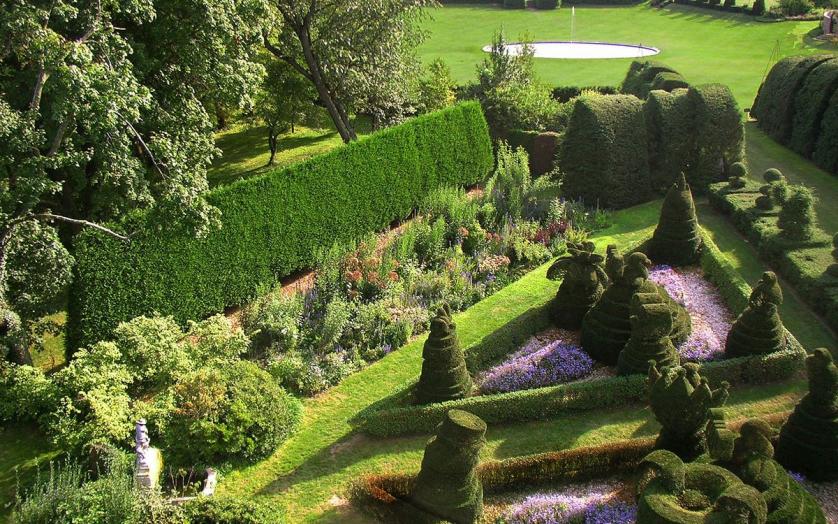This photograph captures a meticulously manicured garden from a high vantage point. In the top left corner, a cluster of tall, pale green leafy trees forms a natural border. Below these trees to the right, a lush checkered lawn expands, punctuated by a simple, bright fountain emitting a single stream of water. Adjacent to the lawn on the left, a smooth, bright green hedge curves slightly leftward, its considerable height emphasizing its prominence.

To the right of the hedge stretches a line of neatly trimmed, tall, rounded wedge-shaped bushes. At the base of this hedge, a rectangular garden bed bursts with variety, showcasing pastel flowers and plants in shades of reddish, pink, and green. In the bottom left corner stands a gray statue, its details somewhat obscured but adding a classic touch to the scene.

Just to the right of the statue lies a triangular garden bed enclosed by a short, well-trimmed hedge, featuring intricately shaped bushes. These bushes form tall cones adorned with topiary animals, such as a woman with a dress and headscarf, a duck, a podium, a bunny, a crown, and other whimsical shapes. A mirror image of this garden bed is situated just down and to the right, complementing the symmetrical design.

Walkways delineated by manicured hedges weave through the garden, adding to the elaborate layout. Behind the living walls of shaped hedges, unmanicured trees rise, creating a contrast between the wild and the controlled within this grand, verdant oasis.